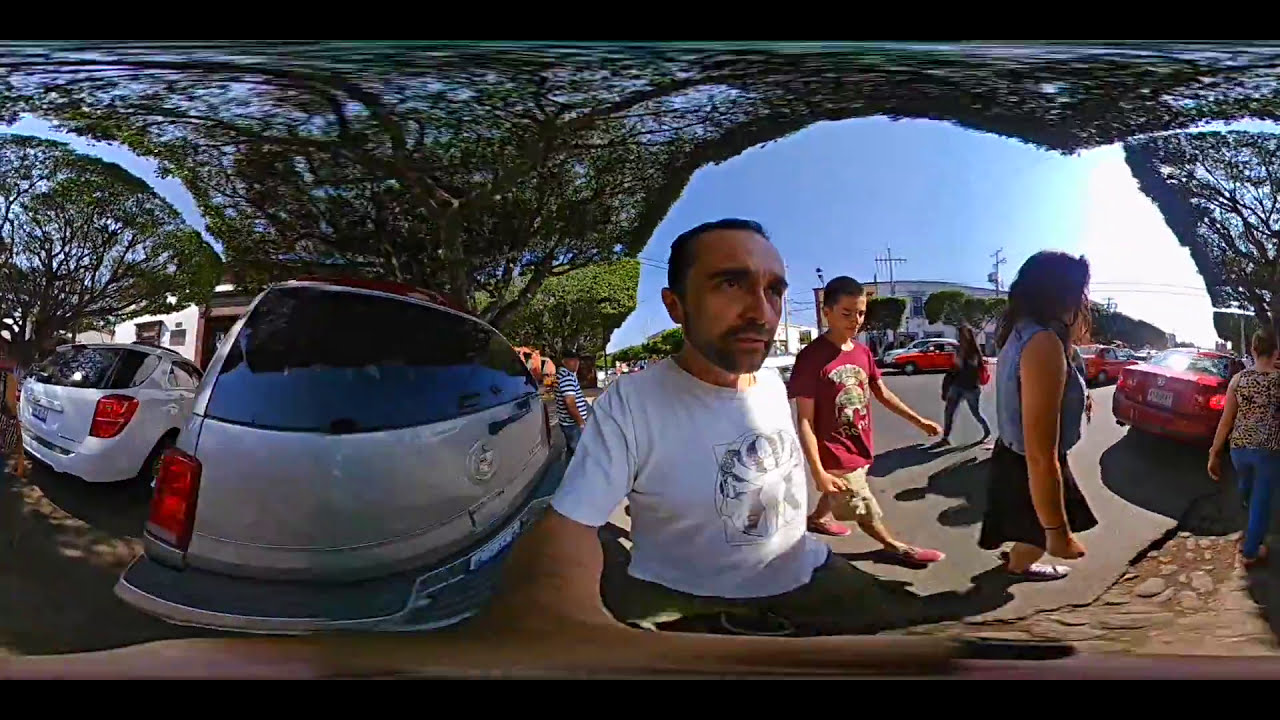The photograph is a color image with a landscape orientation, featuring a panoramic filter that creates a warped, segmented effect. Central to the scene is a man with short black hair, a stubble beard and mustache, wearing a white T-shirt with a black graphic. He has a critical look on his face, and his right arm extends forward, dominating the bottom part of the frame possibly holding a cell phone camera. Surrounding him is a busy and fragmented street scene. 

In the background, to his right, a teenage boy in a burgundy shirt and tan shorts is walking, followed by a woman wearing a black skirt, and another woman in a blue outfit. Behind them, a row of red cars, random people, and a white building are visible. On the left side of the image, there are two parked vehicles - the back of a silver car next to a white one, both near a large tree. The scene is circled with greenery, adding a touch of nature to the urban setting. The combination of disparate elements and warped perspectives gives the photograph a unique, almost surrealistic look.